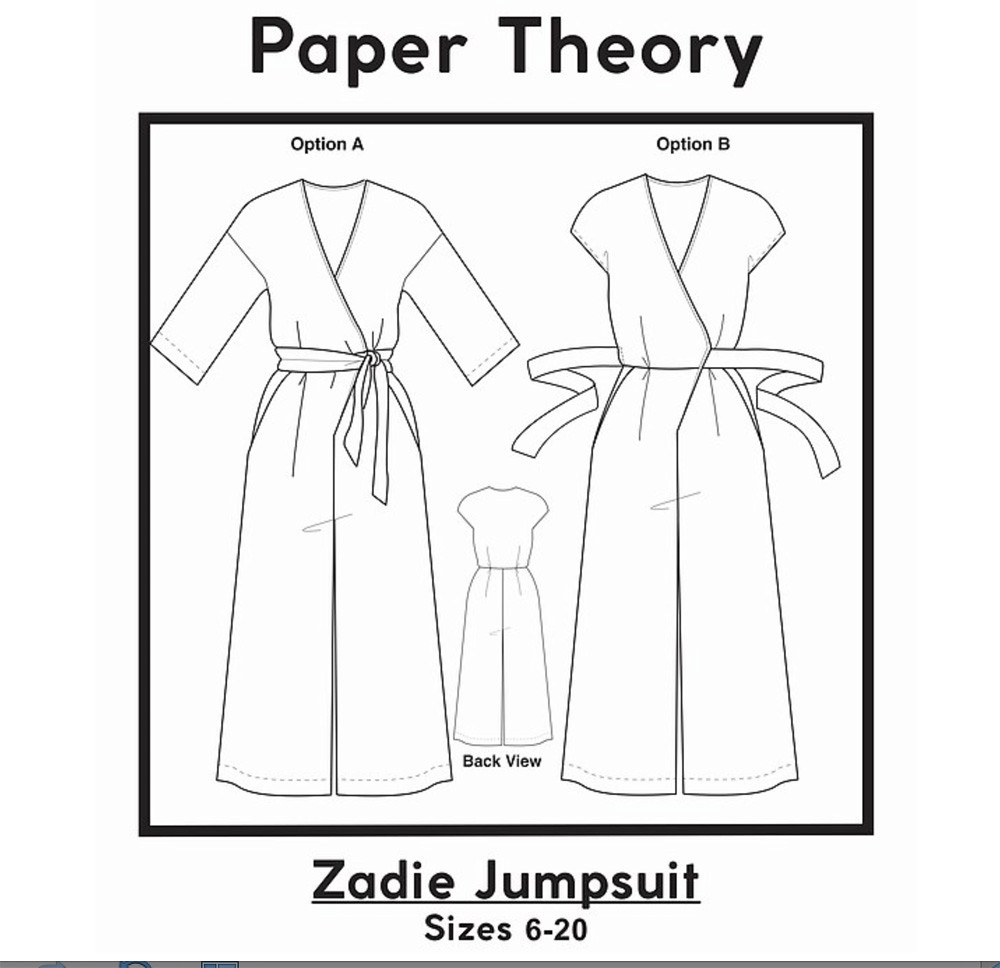The image is a detailed black and white drawing set against a white background, featuring a monochromatic and textile-oriented design. At the top, the heading reads "Paper Theory," followed by a black-outlined square containing three detailed drawings of a jumpsuit. The left drawing, labeled "Option A," shows the jumpsuit with a tied belt. The right drawing, labeled "Option B," depicts the same jumpsuit but with the belt untied. Between these two front-view illustrations, there is a smaller depiction of the back view of the jumpsuit. Below the square, the text "Zadie Jumpsuit" is prominently underlined, with size options ranging from 6 to 20 listed beneath it. This image appears to be an advertisement or design layout for the Zadie Jumpsuit, possibly inspired by paper dolls, underscoring the brand’s emphasis on detailed and structured clothing designs.